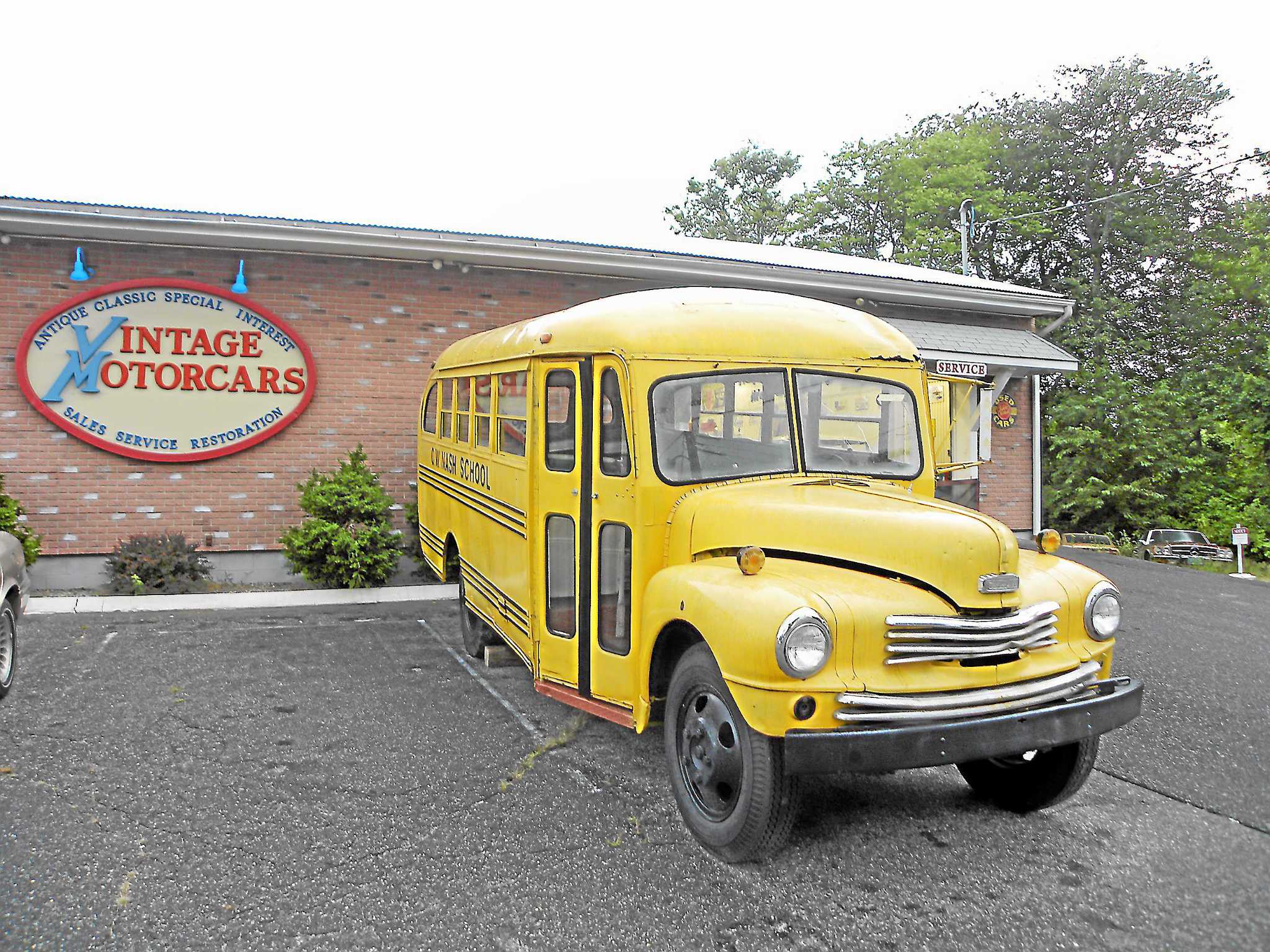The image features a brightly colored, old-fashioned yellow school bus parked in front of a low, brick building adorned with a large sign that reads: "Vintage Motorcars, Sales, Service, Restoration–Antique, Classic, Special Interest Cars." The bus, which appears to be from the 1940s or 1950s, showcases a rounded front with a metal grille and two dome-shaped headlights, with black stripes along its sides. It is smaller than modern-day school buses, evoking a design reminiscent of cars or vans from earlier decades. To the right of the building, there is a door labeled "Service" and another vintage car can be spotted in the background near some trees, adding to the nostalgic atmosphere of the scene.